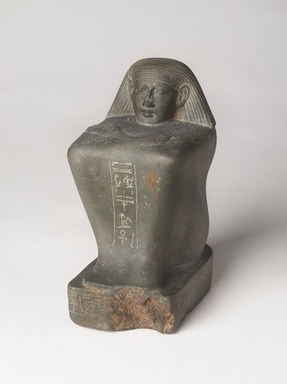The image is a color photograph of a dark gray stone statue believed to depict the Egyptian queen Hatshepsut. The statue features a figure in a seated position, with knees drawn up to the chest and arms crossed in front, resembling a fetal position. The statue's surface is boxy and not highly detailed, with visible hieroglyphics on the front, including the recognizable Ankh symbol. The figure wears a traditional Egyptian headdress and has hair coming down. The base of the statue is a rounded rectangle, but one corner is notably chipped off, revealing a pinkish-brown stone beneath the gray exterior. The backdrop of the image is light blue.